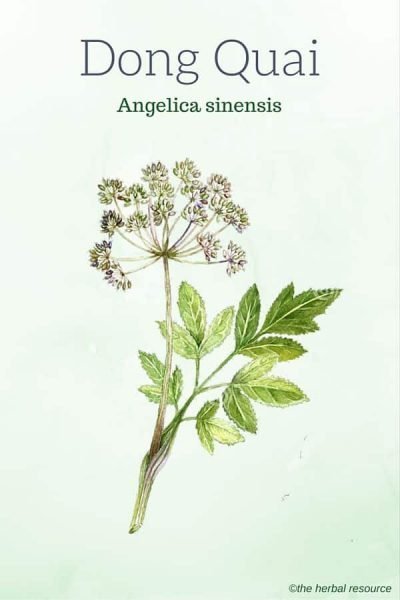This detailed graphic of the medicinal herb Angelica sinensis, commonly known as Dong Quai, displays the plant against a light, pastel blue background with a subtle gradient that deepens to a minty green near the bottom. The image, sourced from 'The Herbal Resource,' prominently features a compound branch showcasing both delicate clusters of cream-colored flowering umbels and distinct, three-part oval-shaped leaves with intricate veining. Resembling a refined dandelion in its bloom structure, the ethereal flowers have a fan-like appearance. The overall illustration, not a photograph but a meticulous drawing, conveys an elegance and clarity designed to reflect the botanical's characteristics. Engraved at the bottom right is a copyright symbol certifying its connection to 'The Herbal Resource,' while the plant's identification is labeled at the top as Dong Quai Angelica sinensis.